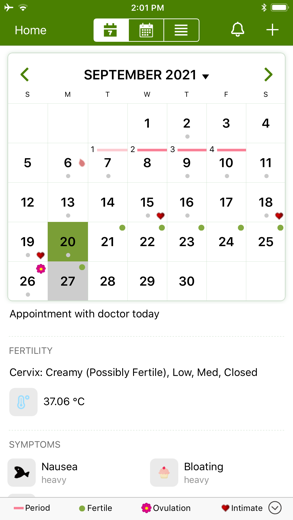This image features a screenshot of a smartphone displaying an ovulation calendar app for September 2021. At the top of the screen, a green background houses essential icons: the time is 2:01 PM, with the Bluetooth and badge icons visible on the top right, and the Wi-Fi and flight mode icons on the top left.

The app provides a detailed overview of fertility and menstrual cycles. The period spans from September 1st to 3rd, marked with a red line. Fertility days are indicated by green dots and occur from September 20th to 27th, with ovulation specifically on the 26th, symbolized by a pink flower. Intimate days, represented by hearts, are noted on the 15th, 18th, and 19th.

Additional information includes an appointment with a doctor today, and various health metrics and conditions: extreme possible fertility, safe periods, no medication (meds) closure, and a recorded basal body temperature of 36.07°C. Symptoms logged are heavy nausea and bloating.